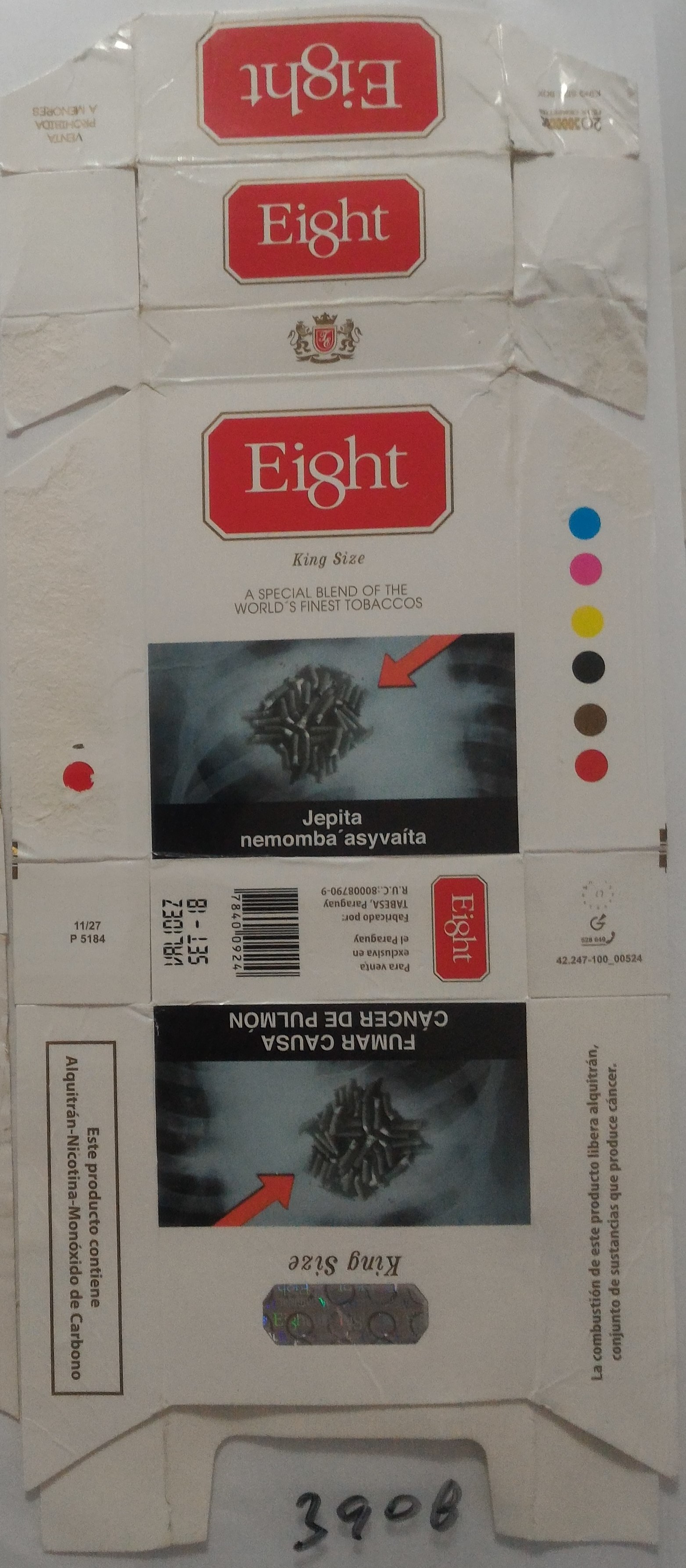The image showcases a carefully deconstructed tobacco product packaging that is laid flat, revealing all its details. The box, once a closed structure, is now opened and spread out, with all flaps and edges entirely unfolded. The brand name displayed prominently across multiple sections of the package is "Eight," creatively spelled "E-I-8-H-T" to give it an elegant touch. 

The packaging features a red medallion logo with a white frame and eight sides, inside of which the word "eight" is printed in white letters. The text on the side and front of the box advertises it as "King Size" and highlights it as "a special blend of the world's finest tobaccos." Additionally, non-English text resembling a health warning is present, reading "F-U-M-A-R C-A-U-S-A C-A-N-C-E-R D-E P-U-L-M-O-N," alongside an image of a chest X-ray with cigarette butts and a red arrow pointing to them, indicative of a government-mandated health warning.

The packaging includes several technical details such as a bar code located on what would have been the bottom of the pack, the same "Eight" logo, and some upside-down text. There is also a test spot featuring colored dots (blue, pink, yellow, black, brown, and red) used by the printer to confirm the accuracy of the ink colors used in the packaging. Lastly, prominently written in magic marker at the bottom center is the collectible number "3908."